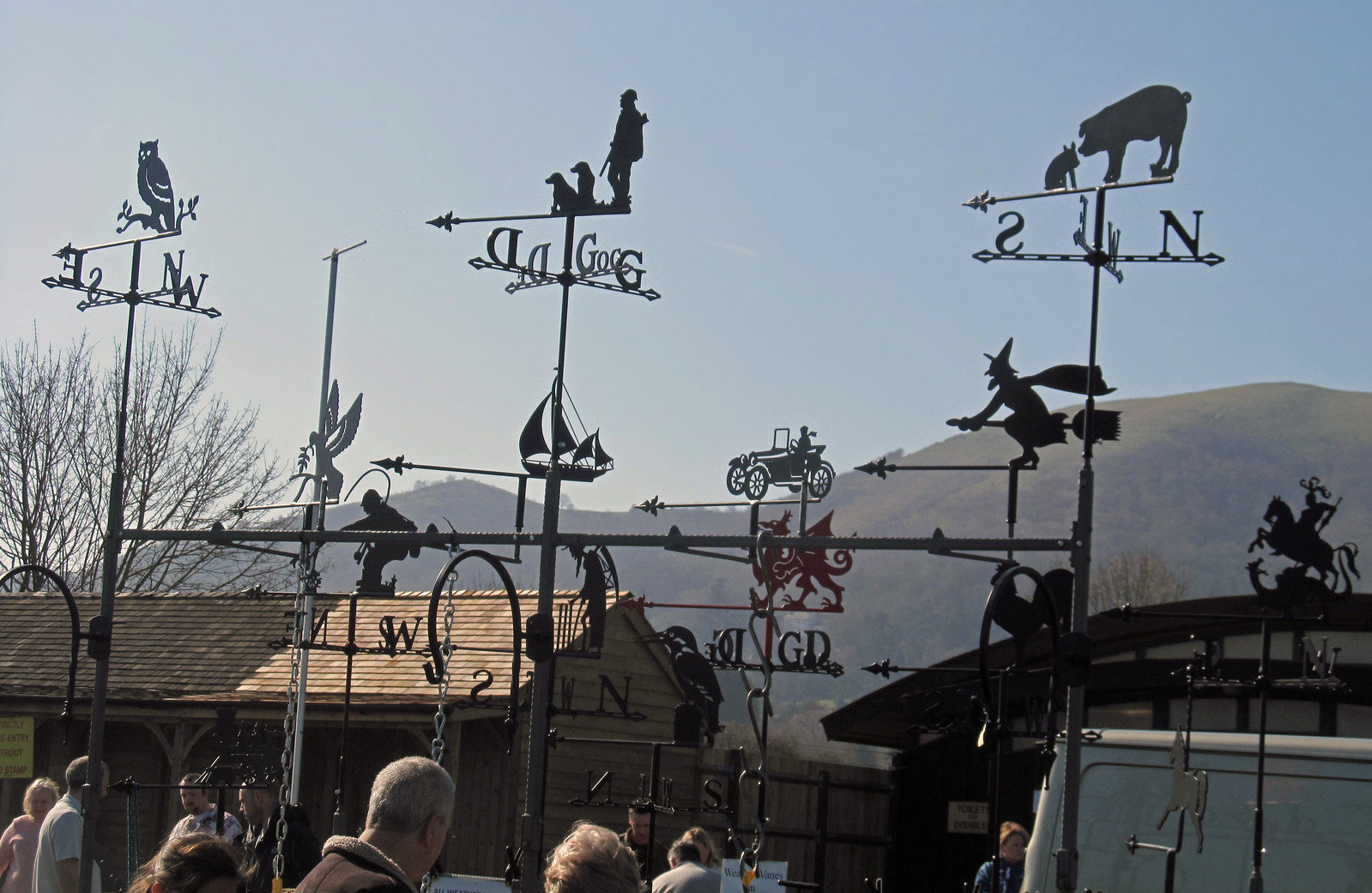This photograph captures a vivid outdoor scene showcasing a collection of wind direction devices, commonly known as weathervanes. The photo appears to be taken at an open show or fair held during the daytime under slightly overcast skies, with green rolling hills and rustic buildings providing a picturesque backdrop. 

The weathervanes are crafted from sheet metal and are mounted on black metal rods with crossbars, each displaying the cardinal directions: North, South, East, and West. They are intricately designed with various motifs, including popular ones like two pigs, a witch, an owl, a dove, sailboats, and dogs—some of which are accompanied by whimsical phrases like "Good Dog." The devices are clustered around a central pole, creating a striking aerial display. The photograph is taken from an upward angle, allowing a glimpse of people in the background, albeit mostly from the shoulders up, adding to the bustling yet charming atmosphere of the event.